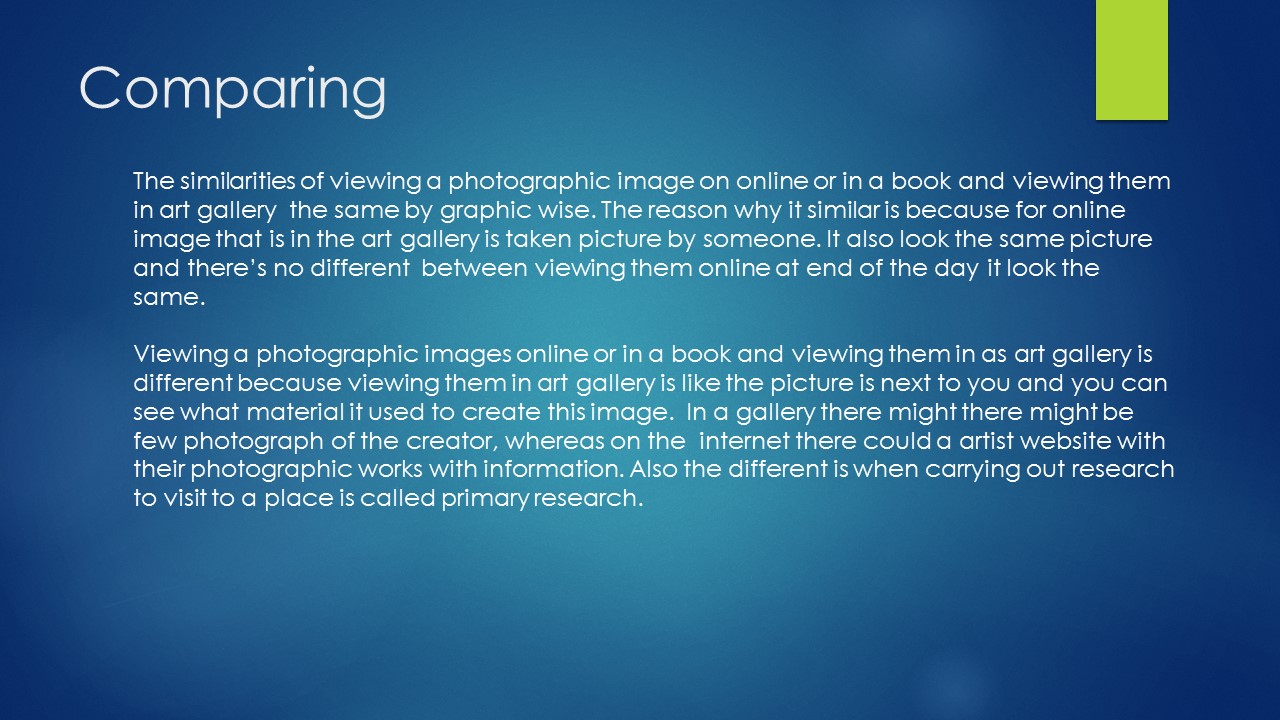The image is a slide from a slideshow, featuring a dark blue background with a slightly brighter spot in the middle. There is a large green bookmark-like shape in the upper right corner. The main text in white font reads: "Comparing the similarities of viewing a photographic image online or in a book and viewing them in an art gallery." The slide explains that viewing an image online or in a book is similar to seeing it in an art gallery because, in both cases, the image was taken by someone and appears the same. However, the explanation highlights a key difference: in an art gallery, the photo feels more immediate, allowing viewers to appreciate the materials used to create it. Additionally, while an art gallery may display a few of the creator's works, online platforms or artist websites often offer a broader selection of the artist's photographic works with accompanying information. The slide also mentions the concept of primary research when visiting a place to observe art firsthand. The language on the slide is somewhat awkward, suggesting that English might not be the writer's first language or that it might have been written by a child.